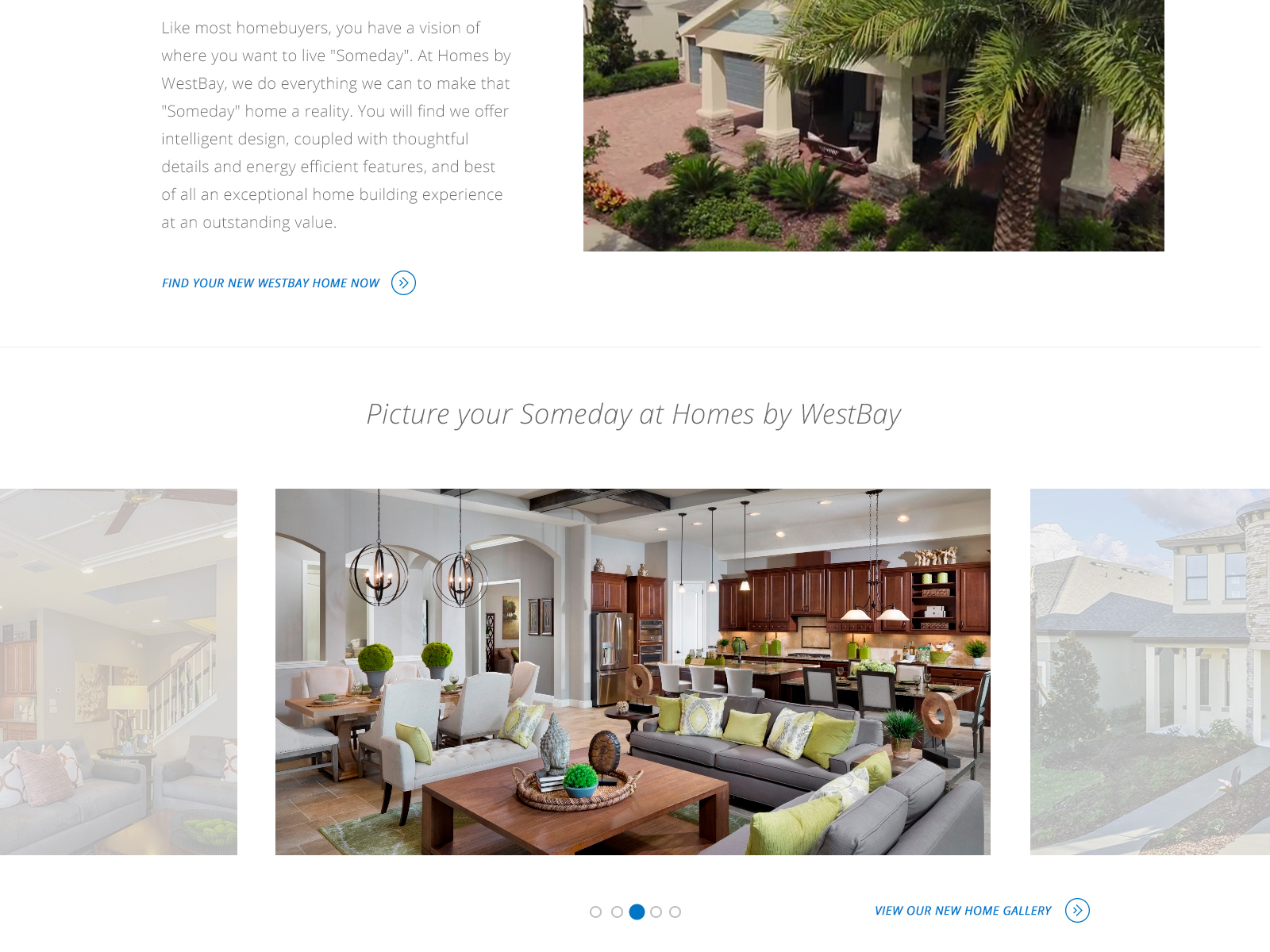Experience Your Dream Home with Homes by Westby

Like most homebuyers, you have a vision of where you want to live someday. At Homes by Westby, we strive to turn that vision into reality. We offer intelligent design combined with thoughtful details, energy-efficient features, and above all, an exceptional home-building experience at outstanding value. 

In the featured image, find your new Westby home with a unique blueprint. The construction site shows a foundation with cement laid out on the ground. To the right, there is a patch of dirt surrounded by green bushes and a towering palm tree. The home itself is aesthetically pleasing with blue wooden exteriors and white pillars, framed by neatly trimmed hedges.

Inside, picture your someday at Homes by Westby. The interior displays cozy sophistication with grey couches adorned with decorative pillows. Overhead lights add a warm glow to the setting, while wooden baskets enhance the rustic charm. In the backdrop, a table and brown cabinets contribute to the overall homey atmosphere. 

Enhance your vision—view our new home gallery. Navigate through with the buttons and arrows provided, and embark on your journey to owning a Westby home today.